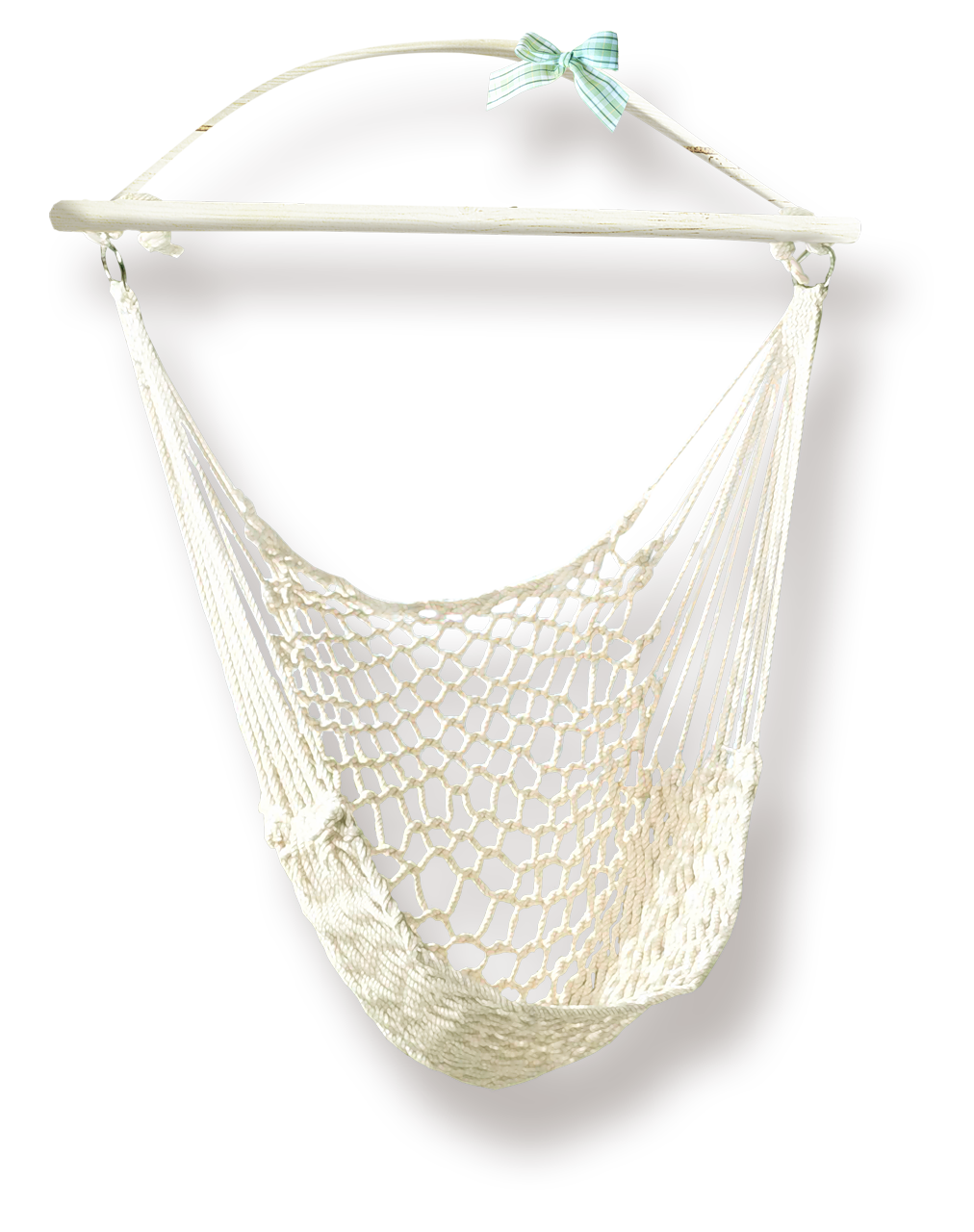This image depicts a white net chair, possibly handcrafted using techniques like macramé, set against a featureless white background. The chair is centered in the frame, and at the top, an arched structure, resembling a wicker design, supports the piece. Just above the right side of the arch, a decorative green bow, made from what seems to be ribbon, adds a touch of color. The arch is connected to a horizontal white board below it, which features two silver round hooks.

These hooks anchor the intricate white netting that forms the chair. The netting consists of numerous straight threads that descend diagonally towards the center and then transition into circular patterns in rows. This design creates both the backrest and seat area, providing a unique and artistic place for someone to sit.